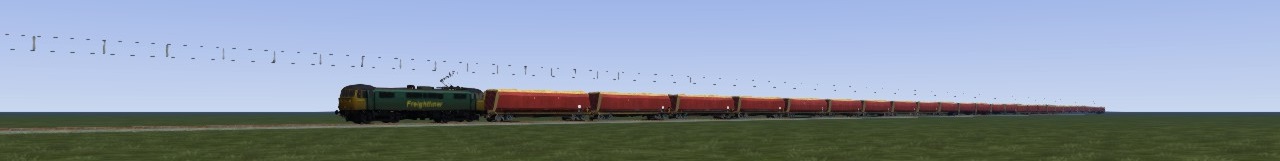This image is a digitally generated panoramic photograph showcasing a lengthy train traveling across a flat, green landscape. The photograph is oriented horizontally and is significantly longer than it is tall. The train, composed of a dark teal locomotive with yellow accents and many identical red cars, stretches from the foreground into the distant horizon, spanning the width of the image. The red cars each feature a small yellow mark towards the back, and they follow the same grayish-brown track that diagonally traverses the green grass, cutting through the lawn from the upper left-hand side to the bottom right-hand side of the image. A series of short, spotty black lines, resembling a telephone wire, runs above the train and becomes harder to discern further back due to the angle. The clear blue sky overhead is devoid of clouds, contributing to the crisp and uninterrupted nature of the scene.